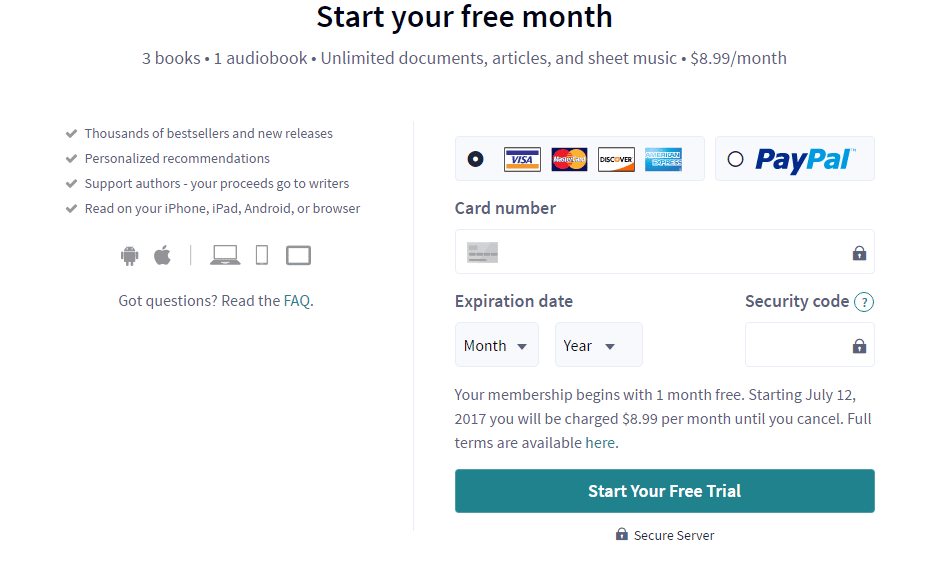A computer screenshot displays a subscription sign-up page with a predominantly white background. At the top center, prominently bolded in black text, it announces, "Start Your Free Month." Two lines below, centered in gray text, it lists the subscription benefits: "Three books · One audiobook · Unlimited documents, articles, and sheet music" followed by the price "$8.99/month."

Approximately four lines below, aligned to the left, there are four bullet points in gray text, each beginning with a gray check mark. They list:

1. Thousands of bestsellers and new releases
2. Personal recommendations
3. Support authors – your proceeds go to writers
4. Read on your iPhone, iPad, Android, or browser

Beneath these points, a row of device icons is centered.

To the right of this section, a gray box contains payment information. At the top, logos for Visa, MasterCard, Discover, and American Express are displayed in a line. Adjacent to them is a white circle outlined in black, featuring the PayPal logo in dark and light blue.

Below, there are distinct text fields: "Card Number" in gray, followed by an image of a credit card. The next line, also in gray, prompts for "Expiration Date," with "Security Code" to the right. A circle outlined in green with a green question mark inside is to the right of the "Security Code" prompt. The form requests the month and year of the card's expiration date.

At the bottom of the gray box, there is a green rectangle with white text reading, "Start Your Free Trial."